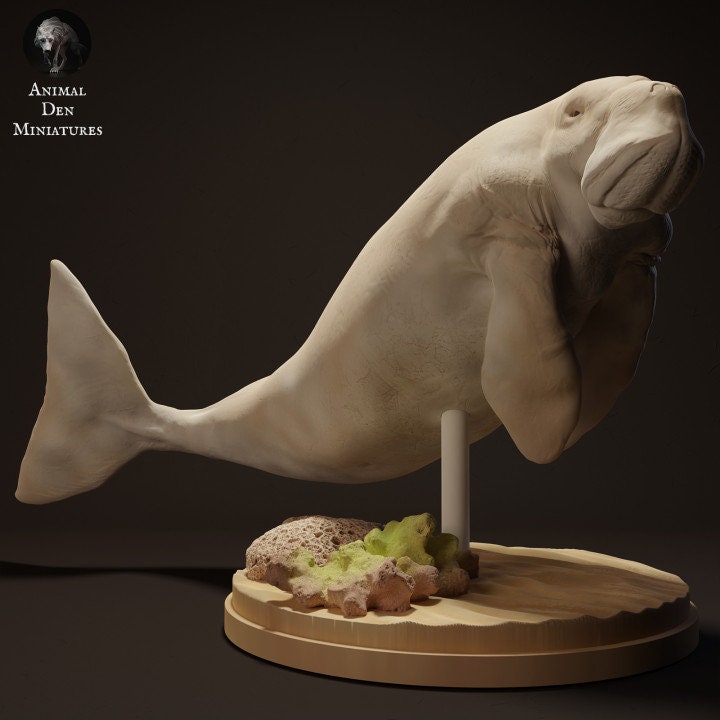The image features a detailed miniature sculpture from Animal Den Miniatures, as indicated by their logo in the upper left corner, which also includes a small wolf icon and the words "Animal Miniatures." The focal point of the image is a lifelike, pale gray manatee statue. This intricately crafted figure is mounted on a circular wooden base, with layers resembling natural seafloor elements such as coral and rocks. The manatee is attached to a white pole that rises from the center of the base, positioning the animal in a dynamic pose as if it is swimming. The manatee's tail points to the left side while its face is angled upward toward the right, offering a sense of motion. The fins are delicately sculpted, pointing downward, enhancing the lifelike appearance of the miniature. The image appears to be professionally lit, possibly for a catalog, to highlight the fine details of the sculpture against a subtly contrasting background.